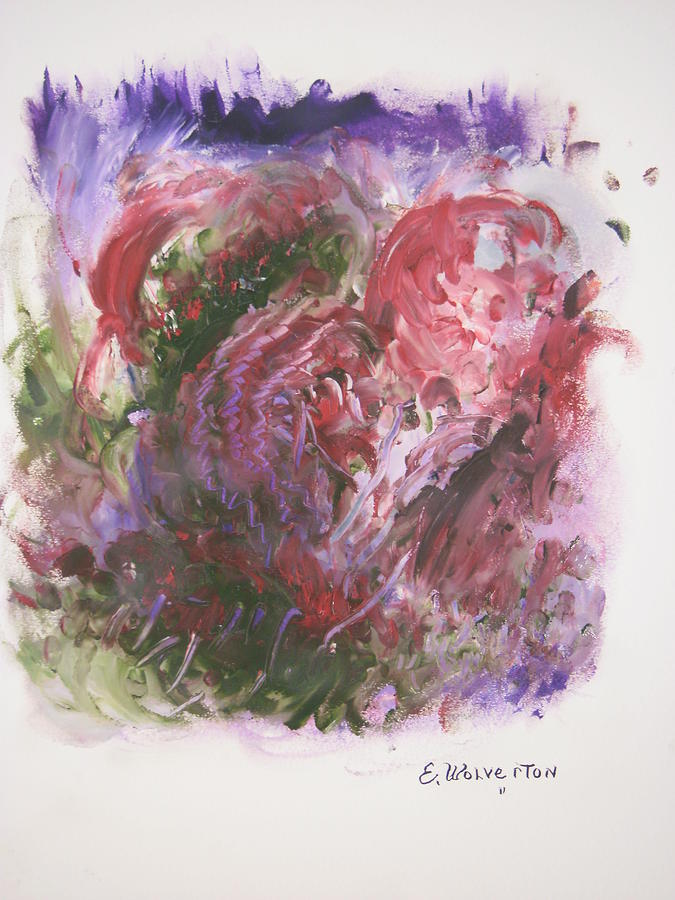This abstract painting by E. Wolverton is done on a white canvas and features bold, impressionistic slashes of color that occupy approximately three-fourths of the canvas, leaving a substantial amount of open white space. The artist's signature is located in the bottom right corner of the image. The composition is dominated by rich purple hues at the top, which blend into swirling masses of reddish pink through the center and the right, resembling erratic smears and chaotic patterns. Small dabs of green are dispersed throughout the middle, with denser concentrations on the left side and towards the bottom. Black accents intermix with the reddish pink on the right side and further integrate into the middle, adding depth and contrast to the vibrant palette. The painting is highly abstract and impressionistic, with thick, expressive brush strokes that give it a dynamic and unrestrained feeling, making the viewer interpretive of its abstract forms and energetic colors.